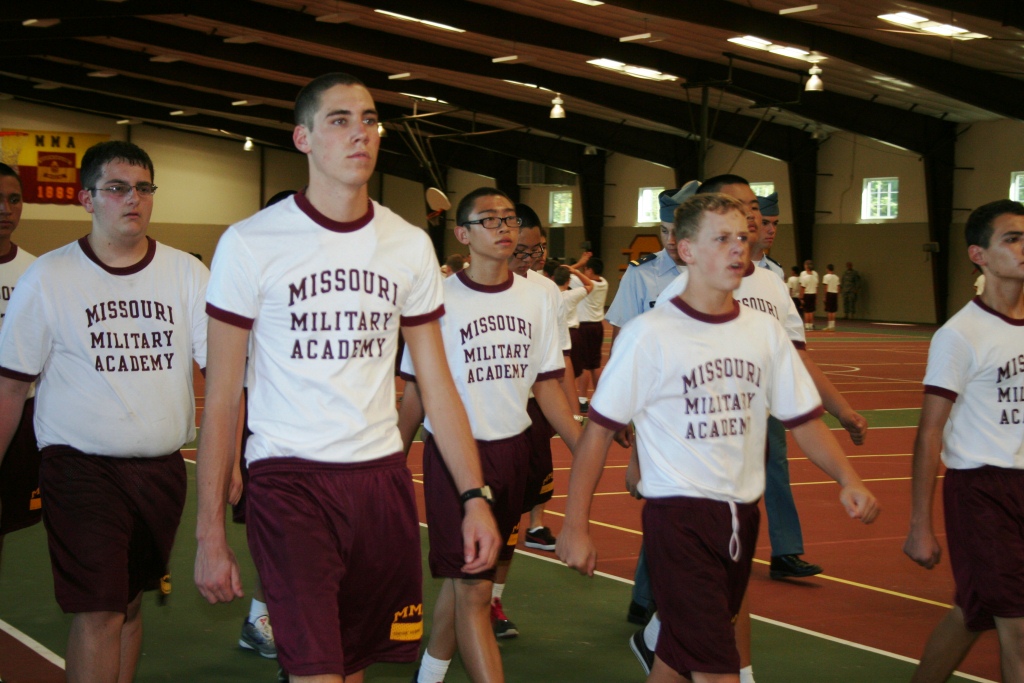This photograph captures a group of cadets, likely teenagers, from the Missouri Military Academy, walking in formation inside an indoor gymnasium. The cadets are dressed uniformly in white t-shirts with burgundy trim and the words "Missouri Military Academy" emblazoned on the front, paired with burgundy shorts, white knee socks, and sneakers. They tread along a green artificial turf segment of the gym floor, which is bordered by a brown track-like area marked with white lines. Behind them, other cadets engage in a basketball game, with hoops visible in the background. The gymnasium itself is expansive, sporting low ceilings, poor lighting, and small windows scattered around, lending a dim atmosphere. The students exhibit a diverse range of ages, races, and heights, and all have serious expressions as they focus ahead. A school logo, though partially illegible, is visible in the background, hinting at a significant historical date.